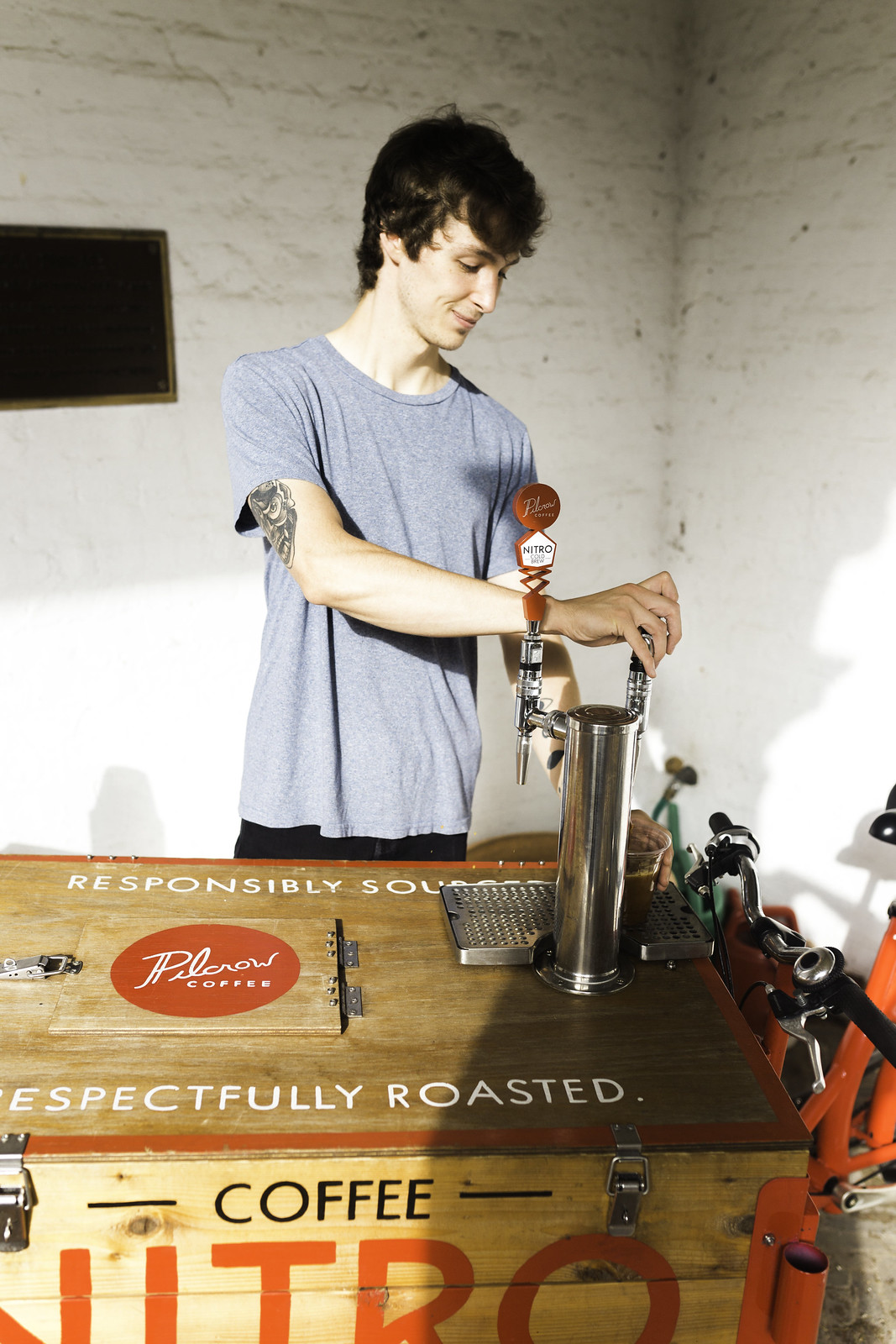The photograph captures a young Caucasian man, likely in his late teens or early twenties, operating what resembles a portable wooden table setup. The focal point of the setup is a brewery tap, which initially suggests it might be for dispensing beer. However, the logos and signage, including phrases like "responsibly sourced" and "respectfully roasted," indicate it is actually for Pilkrow Coffee, possibly serving alcoholic coffee. The scene appears to be in a garage or an outdoor corner of a building, filled with various tools, a bicycle, and some buckets with handles. The young man is engaged in a task similar to pulling a beer tap but is instead producing coffee.